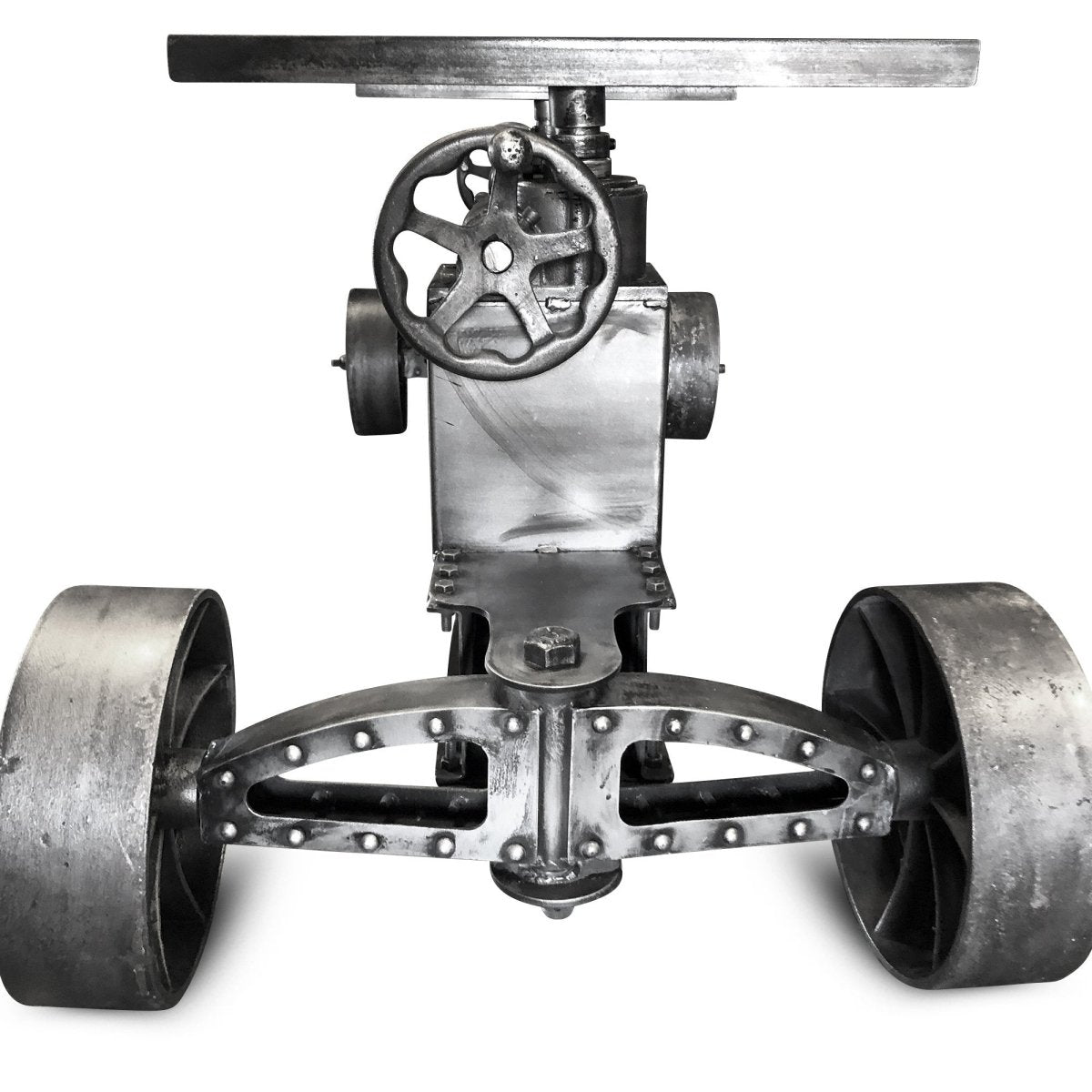The photograph showcases a mechanical device constructed entirely of metal, primarily steel, demonstrating a new yet rustic appearance with visible weld marks and large bolts. The device is set against an immaculate white background, where the wall and floor blend seamlessly. This machinery features a rolling base or trolley with two large, interconnected steel wheels at the front, secured by a prominent rivet and screw. Metal arcs over these wheels, forming a sturdy structure. A flat surface tops the device, above which is a round knob or crank that likely functions to adjust the height or position of a platter or platform at the very top. Additional gears and handles suggest complex mechanical operations, possibly involving the lever mechanism near one of the wheels. Despite the ambiguity surrounding its specific purpose, the intricate design and rugged elegance of this device are striking.